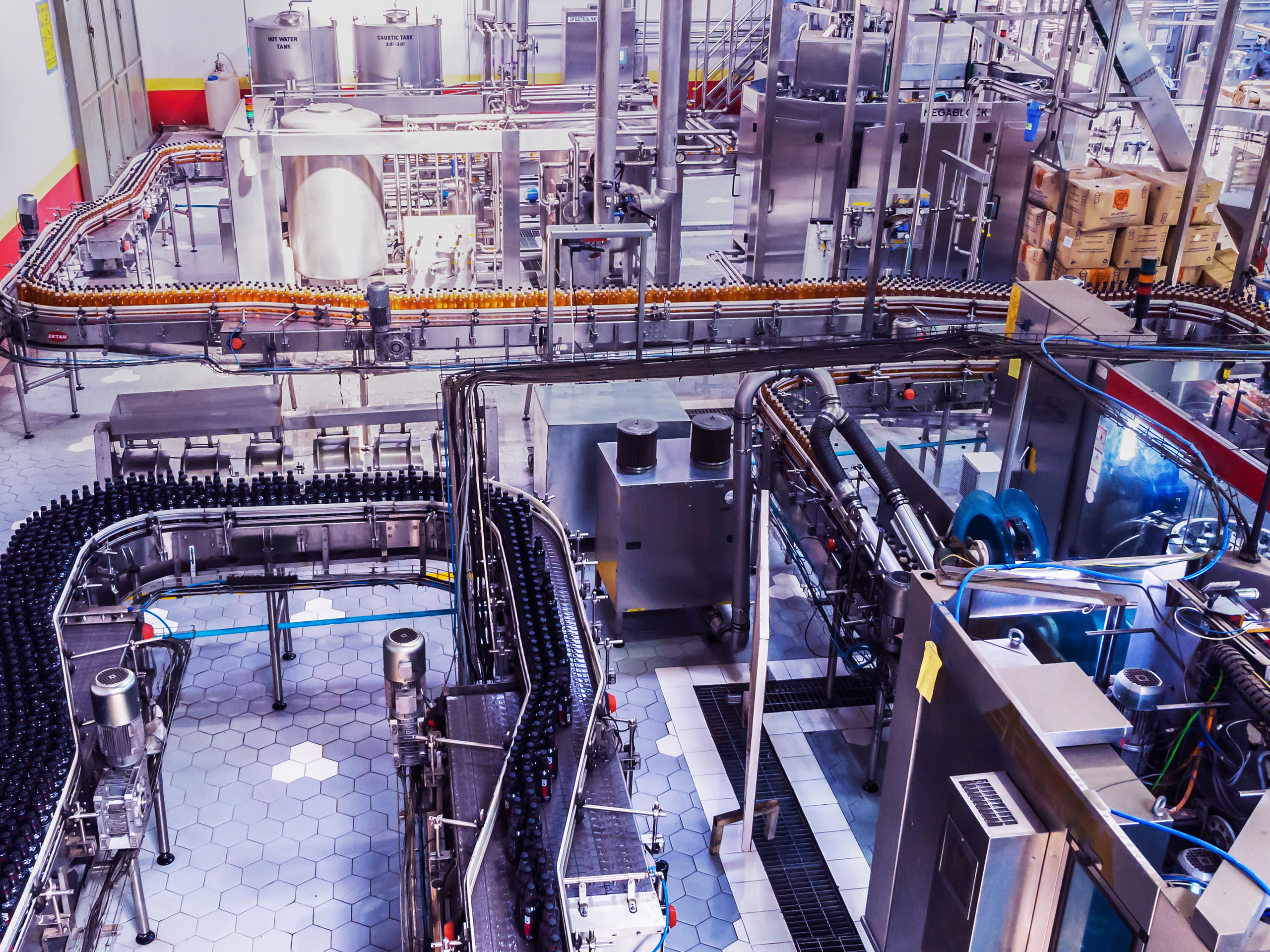The photo captures a vast, well-lit, and impeccably clean bottling facility viewed from a second-floor catwalk or balcony. The floor features a honeycomb white pattern tile, reminiscent of subway flooring, interspersed with several drains. Dominating the scene is an intricate network of shiny stainless steel machinery, including conveyor belts and piping. In the bottom-left corner, a horseshoe-shaped conveyor belt holds numerous bottles, with darker bottles in the foreground and others progressively thinning out to a couple of bottles wide. Parallel, another conveyor belt begins at the far top-left, moving toward the camera before turning right and extending out of the frame. Notable elements include large, gleaming tanks and clusters of stainless steel tubing branching out from the ground. Further back, a large white tank is visible, in addition to bottles containing yellow liquid. Key features also highlight a blue plastic wheel and large cardboard boxes adorned with an orange shield. The pristine white walls are accented with a yellow border at the top and a red base at the bottom, complementing the industrial aesthetic of the facility.